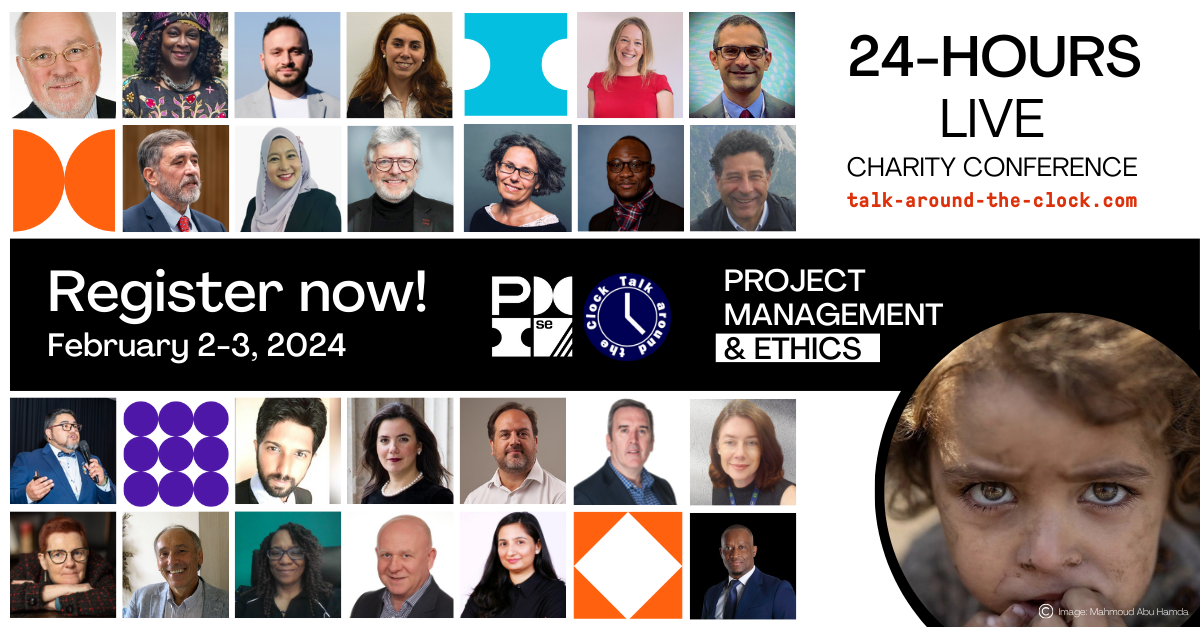Capture the essence of the described image:

---

In the top right corner on a white background, bold black letters announce a "24 Hours Live Charity Conference," with "talkaroundtheclock.com" highlighted in red. A central banner encourages viewers to "Register Now" for an event taking place from February 2 to 3, 2024. The banner features a logo resembling the letter 'P', alongside several indistinct icons. Prominently, "Talk Around the Clock" is creatively scripted in a circular pattern around a clock face. Complementing this, the phrase "Project Management Ethics" is emblazoned across the midsection of the banner.

The top and bottom of the banner are flanked by images of diverse individuals, showcasing a spectrum of races, ethnicities, genders, and ages, most of whom appear older. Interspersed among these photos are colorful background panels that add visual interest. Among the images, near the bottom right of the design, the poignant face of a child, with dirt-streaked cheeks and sad eyes, stands out, adding an emotional depth to the advertisement.

Overall, this visually captivating advertisement blends text, imagery, and color to draw attention to its call for participation in an important charity conference.

---

This detailed caption provides a clear and comprehensive description of the visual elements and the overall impact of the promotional material.